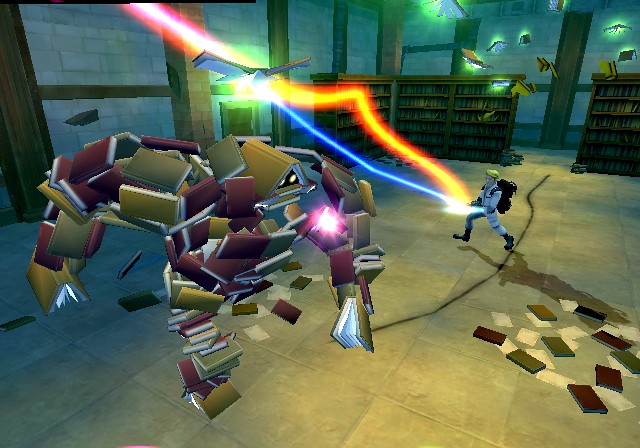This is a detailed, color, computer-generated graphic or screen capture from a Ghostbusters video game. The setting is inside a library, with bookcases lining the background on the far right. Central to the image is a man with blonde hair and glasses, dressed in the iconic white Ghostbuster jumpsuit and black boots. He carries a proton pack on his back, from which he is firing a stream comprising both orange and blue beams that merge into a purple stream, targeting a colossal humanoid monster made entirely out of various books. This book creature, positioned slightly to the left of center, is constructed from rectangular books of tan, brown, and purple hues, with dark yellow circles for eyes. Surrounding the scene, books are scattered on the floor and floating in the air, adding to the chaotic atmosphere. The monster strides towards the foreground and to the right, while the Ghostbuster holds his ground, engaging the creature with his proton stream. There are no visible words or text in the image.